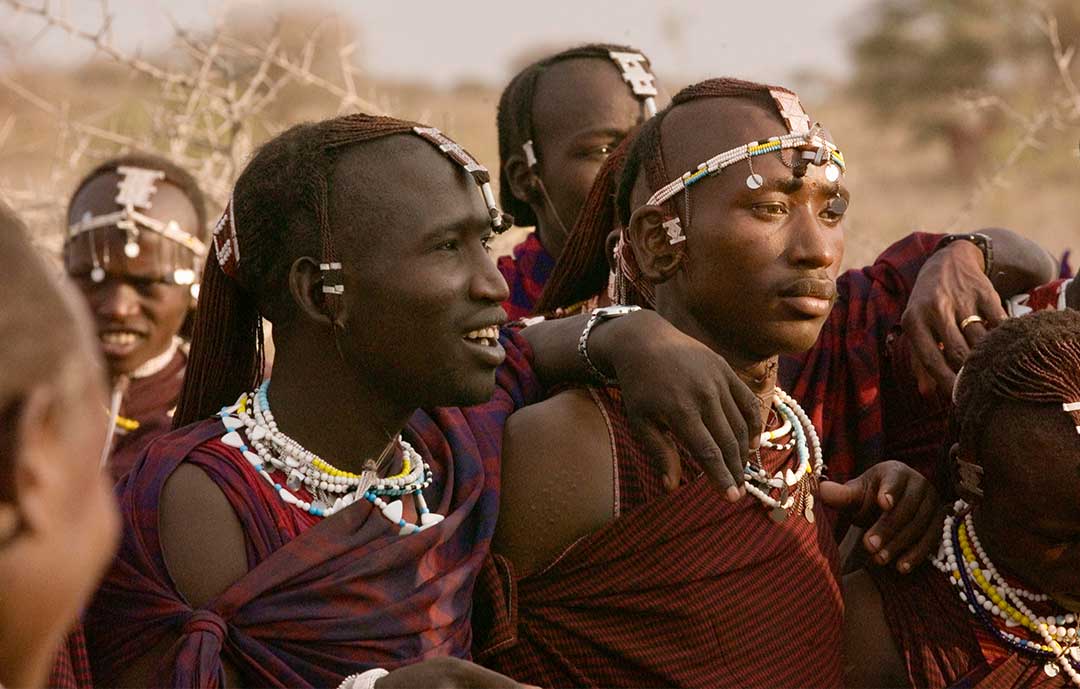The image features a group of six African individuals, likely part of a tribe, gathered outdoors during the daytime. The men and children in the photo have dark skin and are adorned with elaborate headdresses and intricate bead necklaces in a variety of colors including white, green, yellow, blue, and light brown. They are all dressed in red shirts, with some featuring black stripes.

In the center towards the right, a man is seen with a closed mouth, wearing a headband that circles his forehead and a narrow strap that extends over the top of his head. His necklace contains white and light blue beads. Another man, next to him, has his mouth open, revealing his top row of teeth. He wears a band with white and dark brown sections over his head and a collection of colorful bead necklaces. This man has his hand on the shoulder of the man beside him and is wearing a silver watch.

A child is located far to the left; his mouth is open, and he, too, displays a headband. The background is unfocused but shows a grayish-white sky and sparse natural elements with light yellow twigs and a tree with brown branches and green leaves on the top right. The overall scene captures a moment of communal presence and cultural adornment against an indistinct natural backdrop.